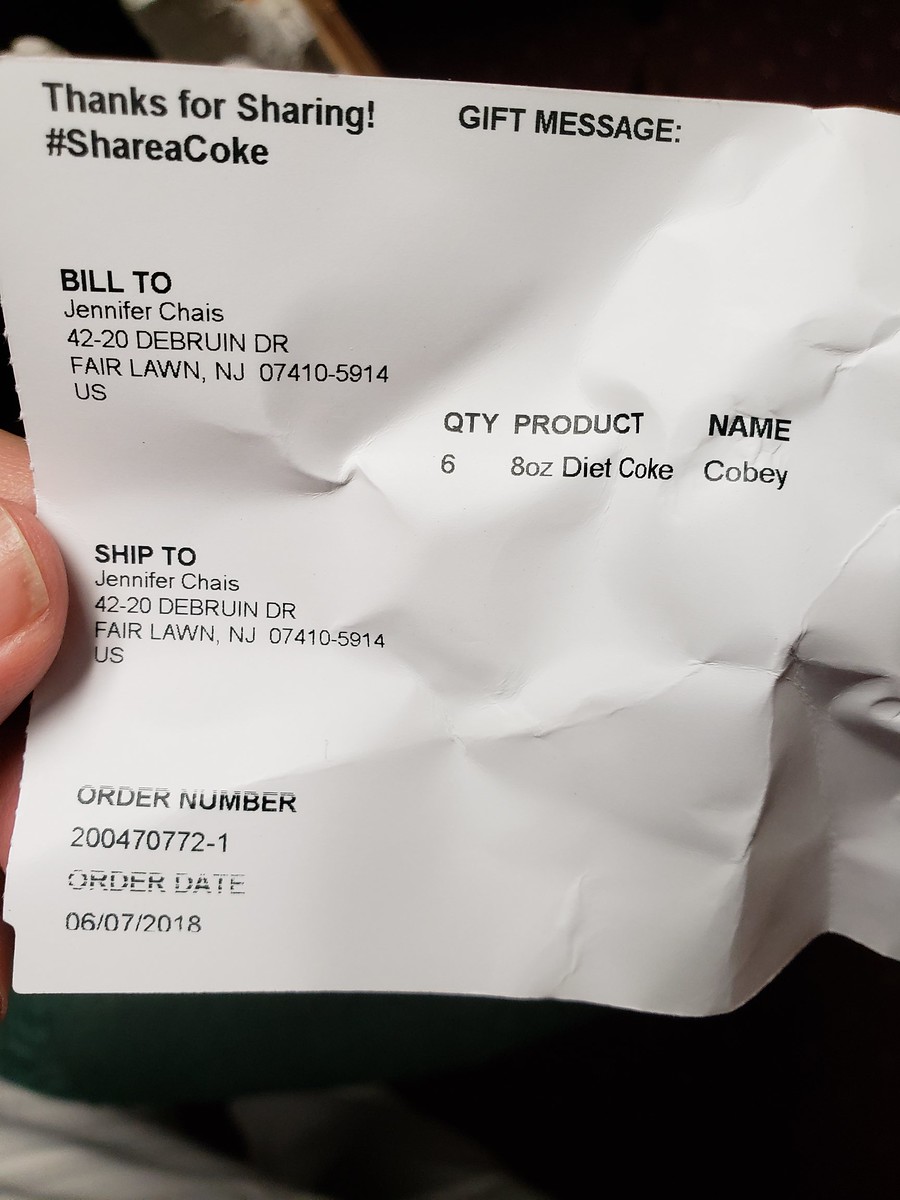This photograph captures a crinkled white receipt held by a person's thumb and finger on the left-hand side, with a mostly black background providing contrast. The black text on the receipt includes a message, "Thanks for sharing, #ShareACoke," followed by a gift message. The receipt is billed to Jennifer Chase at 4220 DeBruin Drive, Fairlawn, New Jersey, 07410-5914, US. It details an order of six eight-ounce Diet Cokes labeled with the name "Kobe." The receipt also includes the recipient's address, which is identical to the billing address. The order number is 040470772-1 with an order date of 6/7/18.